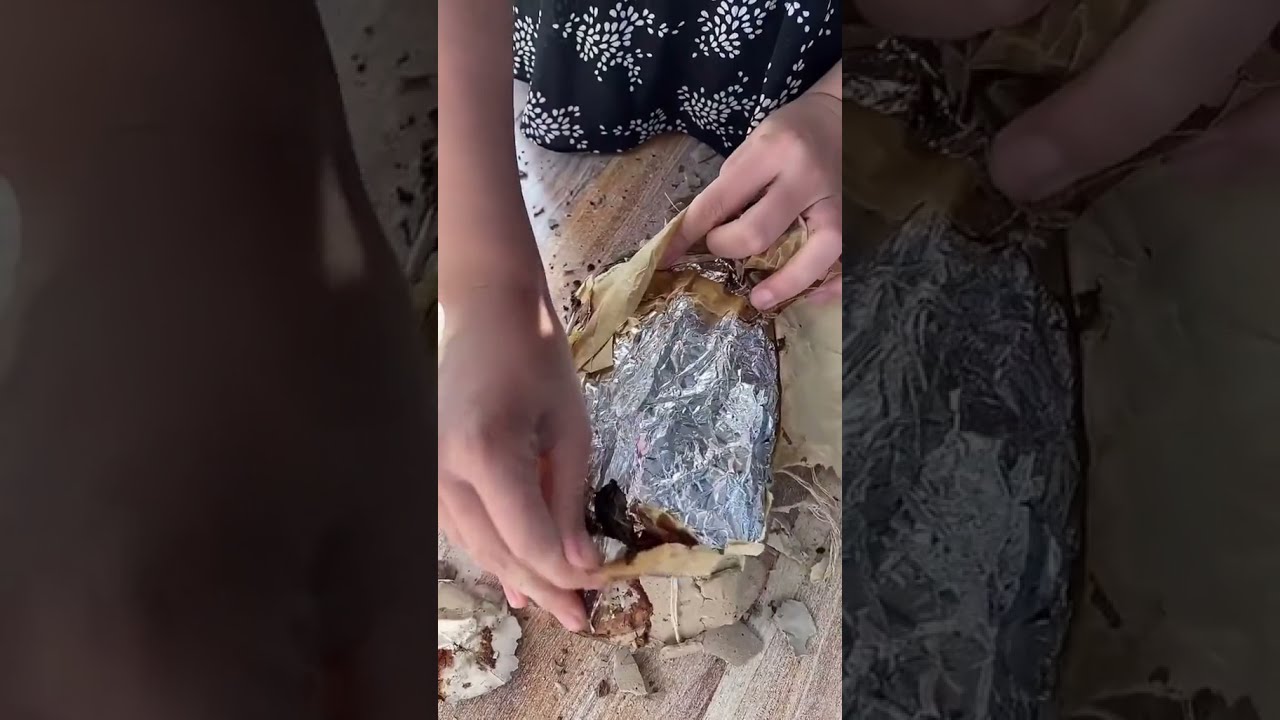This image captures the intricacy of a moment where a young woman's hands are gingerly unwrapping a piece of food encased in silver foil, all set on a light-colored wooden surface. The dark brown food inside suggests it might have been slowly cooked or baked, possibly with a rope-like, tan wrap adding to its rustic appearance. The woman, dressed in a dark blue garment adorned with white leaves, concentrates on unwrapping the foil, with her fingertips and palms gently positioned at the top and bottom of the item, reminiscent of how one might hold a baked potato. Above the scene, a fabric with a black and white dot pattern adds a cozy backdrop. Notably, the bottom left of the image includes a white Chinese bun, neatly split to reveal its rich brown filling, subtly contrasted against the warm tones of the wooden surface. The photo's surrounding edges are darker, enhancing the central activity and making the details of her hands and the wrapped food stand out more vividly.